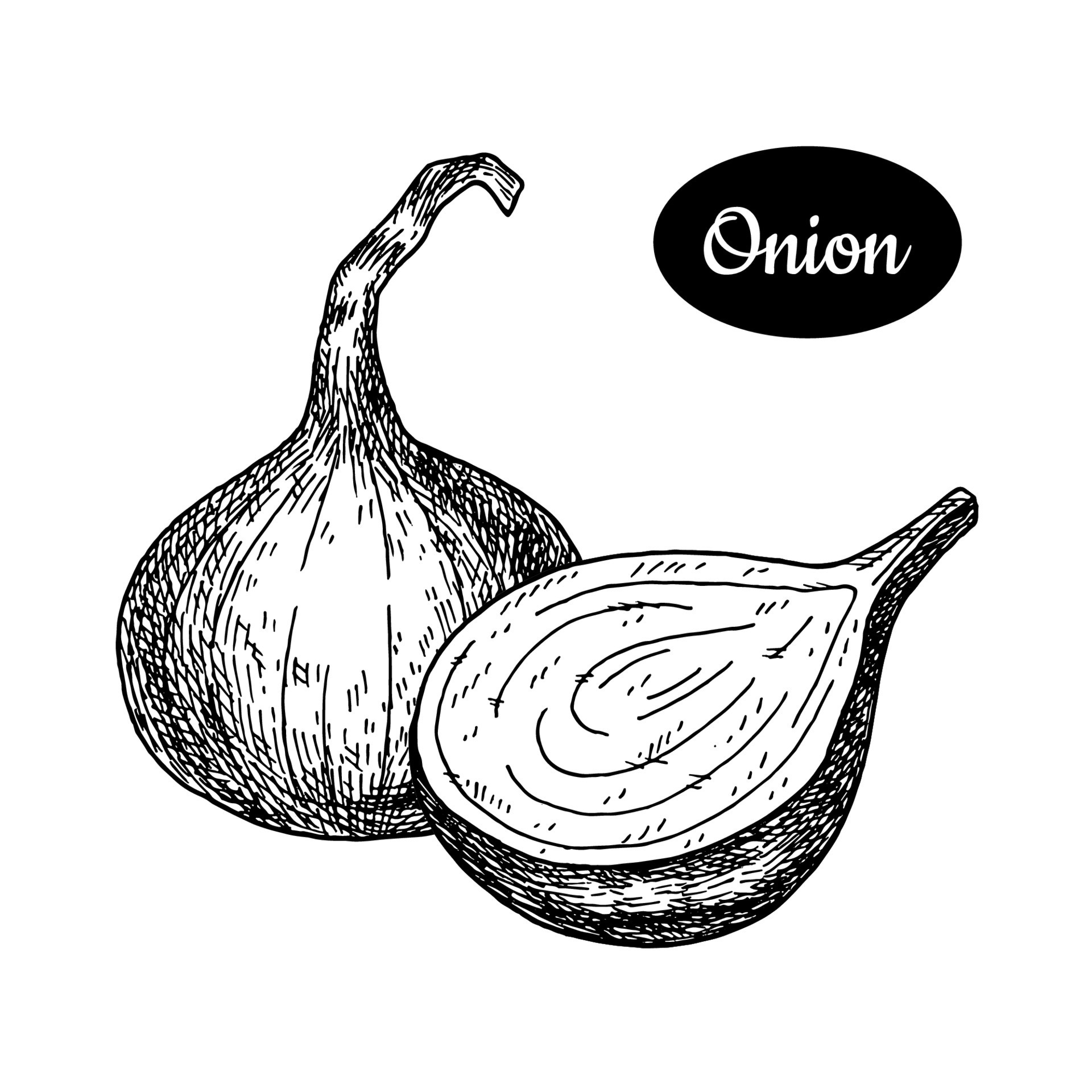This detailed black and white pen sketch features a line art drawing of an onion, showcasing both a whole onion and a half-sliced onion to reveal the inner segments. The whole onion, positioned upright on the left, is detailed with vertical segment lines and cross hatching to indicate its texture and dimensions, complete with a stem at the top. The sliced onion, lying on its back, displays concentric circles to illustrate the inner layers. On the upper right-hand side of the drawing, there's a black oval containing the word "Onion" written in white cursive script, giving it a classic and artistic appeal. The entire artwork is set against a white background, enhancing its clean, minimalist aesthetic, reminiscent of old sketch-style illustrations. This detailed depiction could be an ideal decorative piece for kitchens or promotional material for farmer's markets, enhancing the visibility and appeal of fresh onions.